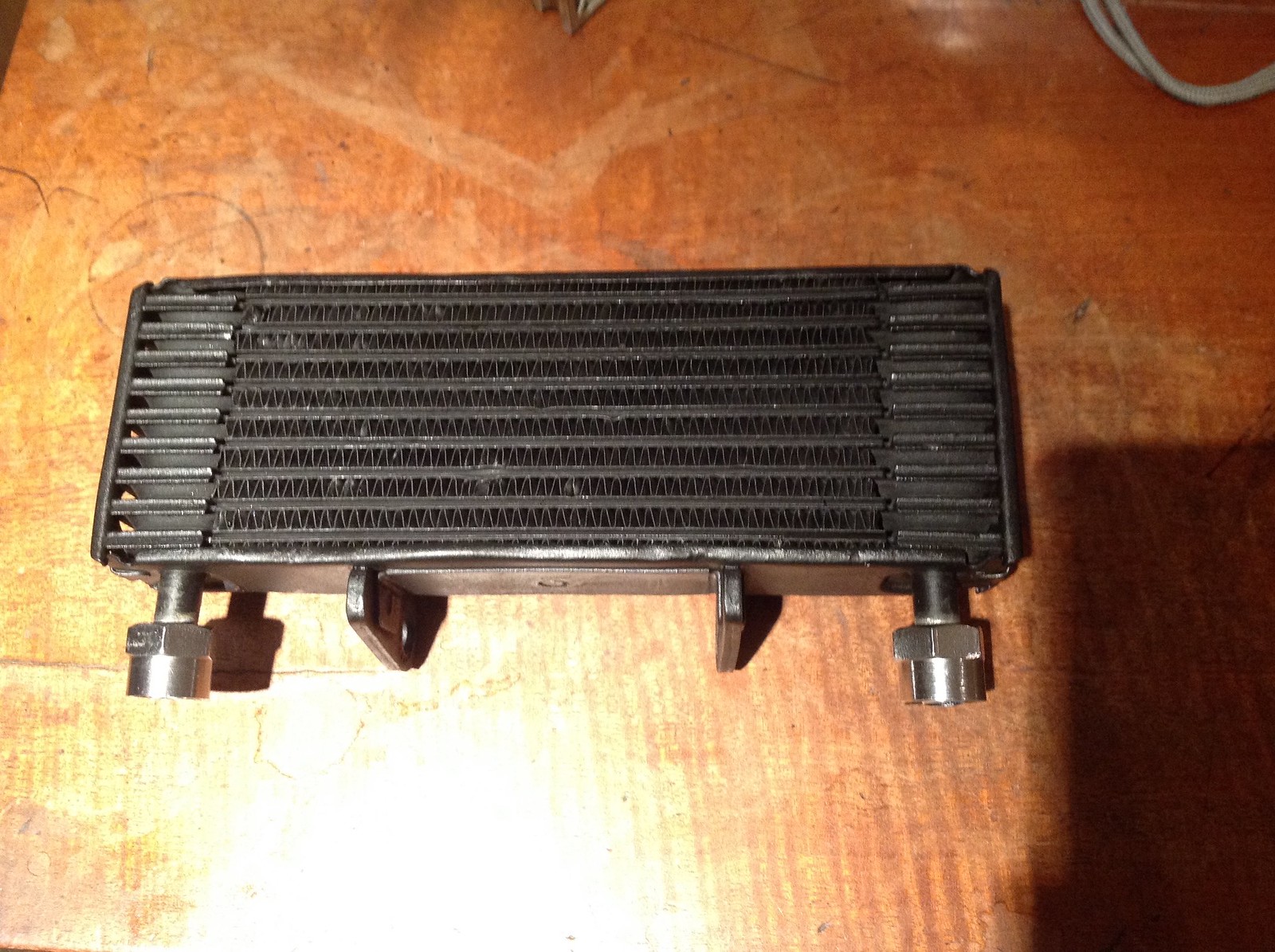The image depicts a detailed close-up of what appears to be a black rectangular condenser or radiator, situated on an old, weathered wooden table. The table, illuminated by a bright light in the foreground, has a noticeable glare that distorts the appearance of its brown wooden surface. The condenser itself features a sleek design with numerous rows of intake and outlet valves, key components for fluid flow. Flanking the ends of the condenser are circular valves with wrench-like claws for secure attachment to hoses or other devices. 

In the central area, a frame with wings and a hole for a potential screw suggests it can be mounted or firmly affixed to a setup. Additionally, metallic bolts and screws can be observed at the bottom, providing structural support and attachment points. This intricate setup comprises a series of crisscrossing lines and pipes, reminiscent of a barbed wire arrangement, adding to the complexity and functionality of this radiator-like apparatus. Intriguingly, some form of marking, possibly a drawn circle, is visible on the wooden floor, adding an element of human interaction with the object.